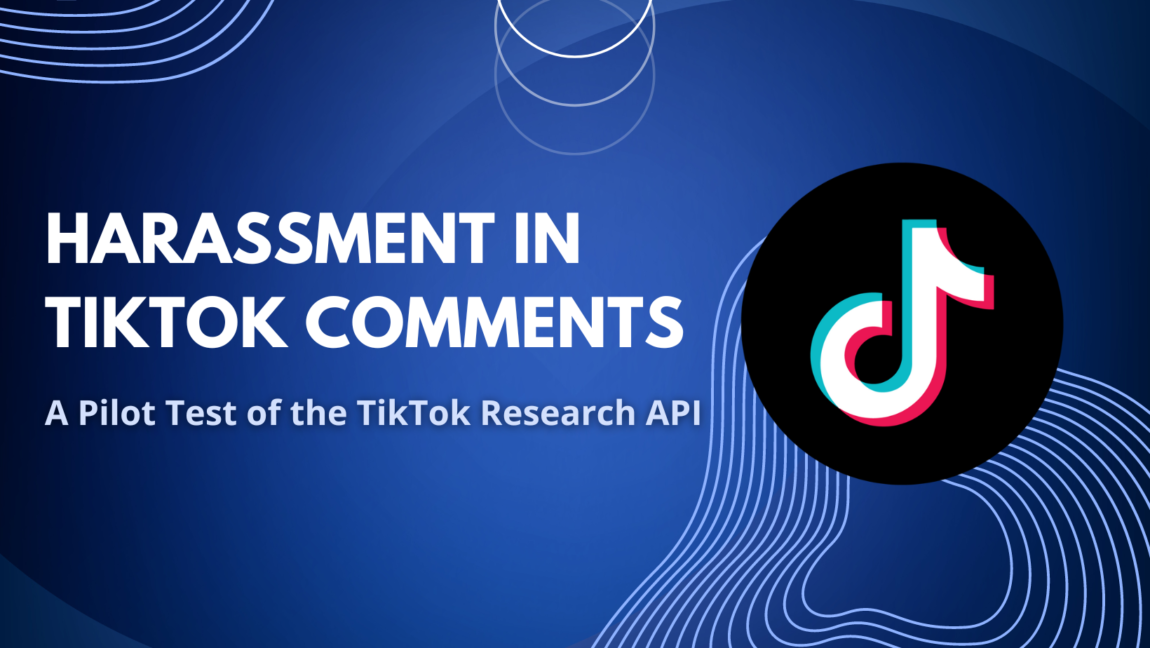This image features a large blue rectangle as its background. In the top left corner, there are lines that form an upside-down rainbow shape. Centered within the image, there are additional lines arranged in half-circle patterns. At the bottom right corner, lines start from the left side of a black circle, curve downward, and then proceed to the right, enveloping the circle partially. The black circle displays the TikTok emblem, characterized by a small TikTok icon inside.

On the left side of the image, bold white capital letters spell out "HARASSMENT IN TIKTOK COMMENTS." Below this text, in light blue, it reads "A pilot test of the TikTok Research API."